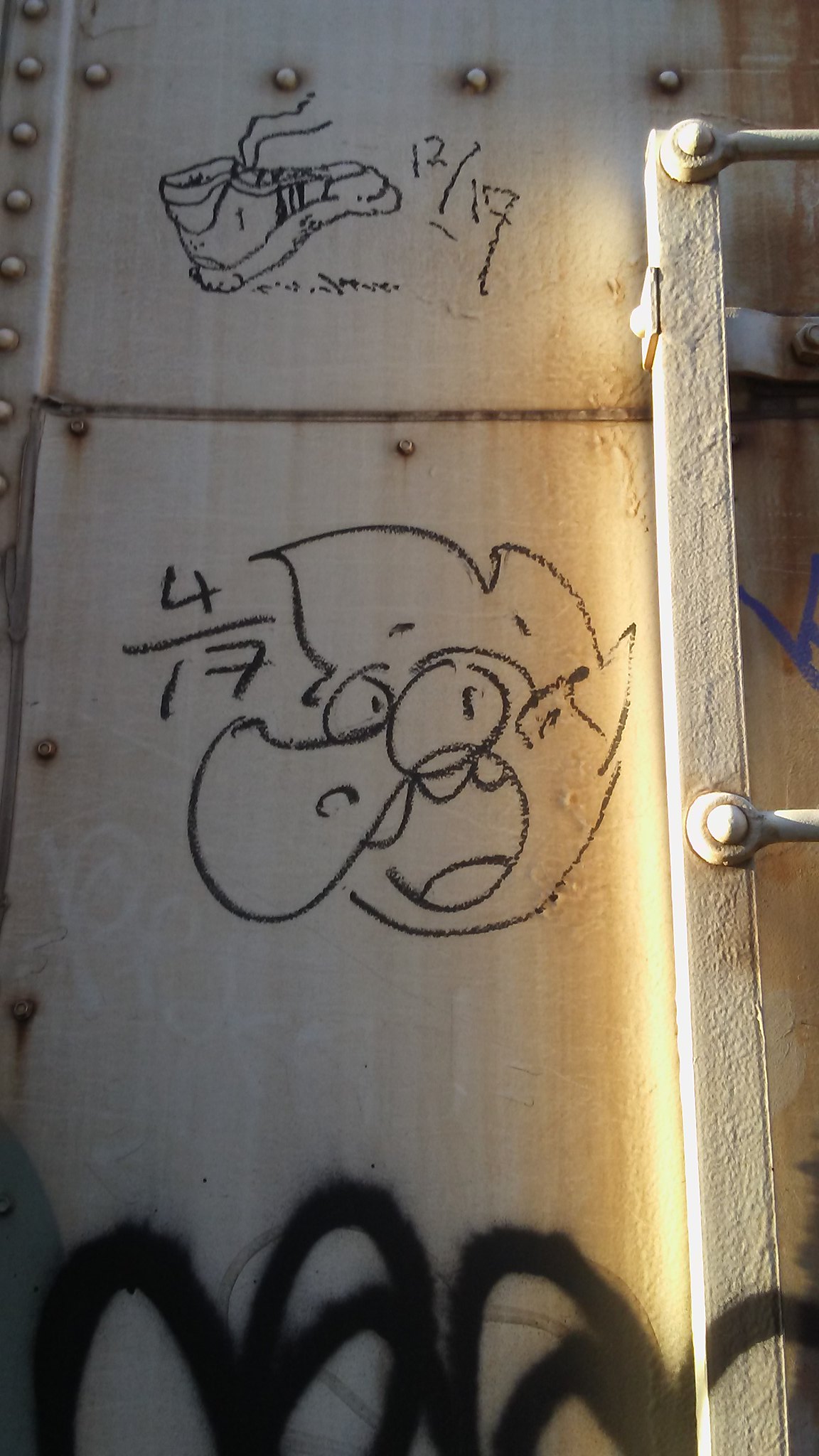Inside a long vertical frame, two tannish metal I-beams are bolted together, creating a cabinet-like structure. The beams are painted white and evoke an industrial feel. At the top, a smaller metal panel is attached, followed by a larger one at the bottom. These panels feature whimsical black graffiti-style drawings, with some numbers seemingly denoting measurements used by a carpenter. On the upper panel, a detailed sketch of a high-top tennis shoe, with its laces flowing outward as if in motion, is placed next to the fraction 12/17. Directly below, on the lower panel, next to the number 4/17, is a caricature of a face with exaggerated features: extremely large eyes, a big nose, bushy hair, and an open mouth showing teeth. The bottom of the image displays graffiti in bold, dark black marker, adding an element of chaos to the constructed arrangement. Light illuminates the horizontal bar attached to the panels, emphasizing the contrast between the industrial background and the creative expressions upon it.